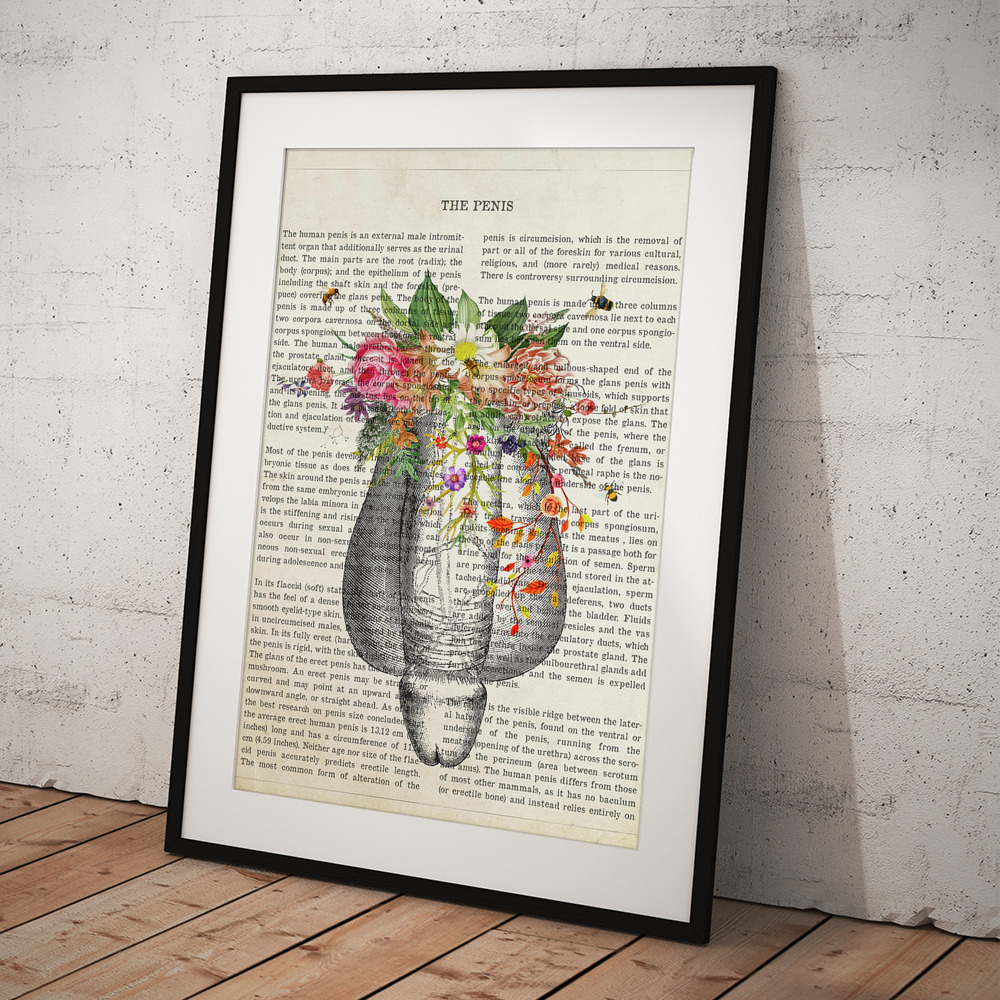The image depicts a full-color photograph of a multi-color print piece, framed in black and leaning against a white-painted, concrete or stone wall. It is staged indoors under artificial lighting. The photograph extends vertically with no visible background beyond the immediate setting. The frame encloses a white mat that surrounds an off-white vertical rectangular poster. At the top of the poster, in black letters, it reads "The Penis," followed by two long columns of black text comprising multiple paragraphs, appearing to be an ode to the male organ. Dominating the center of the poster is a grayscale image of a prominently veined penis with a scrotum behind it. Emanating from the top of the penis and scrotum are vibrant, colorful flowers in shades of pink, red, purple, yellow, and green leaves. The framed piece rests on a brown, slatted wooden shelf or possibly a floor made of light brown or beige wooden planks, slightly angled downward to the left, and facing the camera directly with a slight leftward tilt.